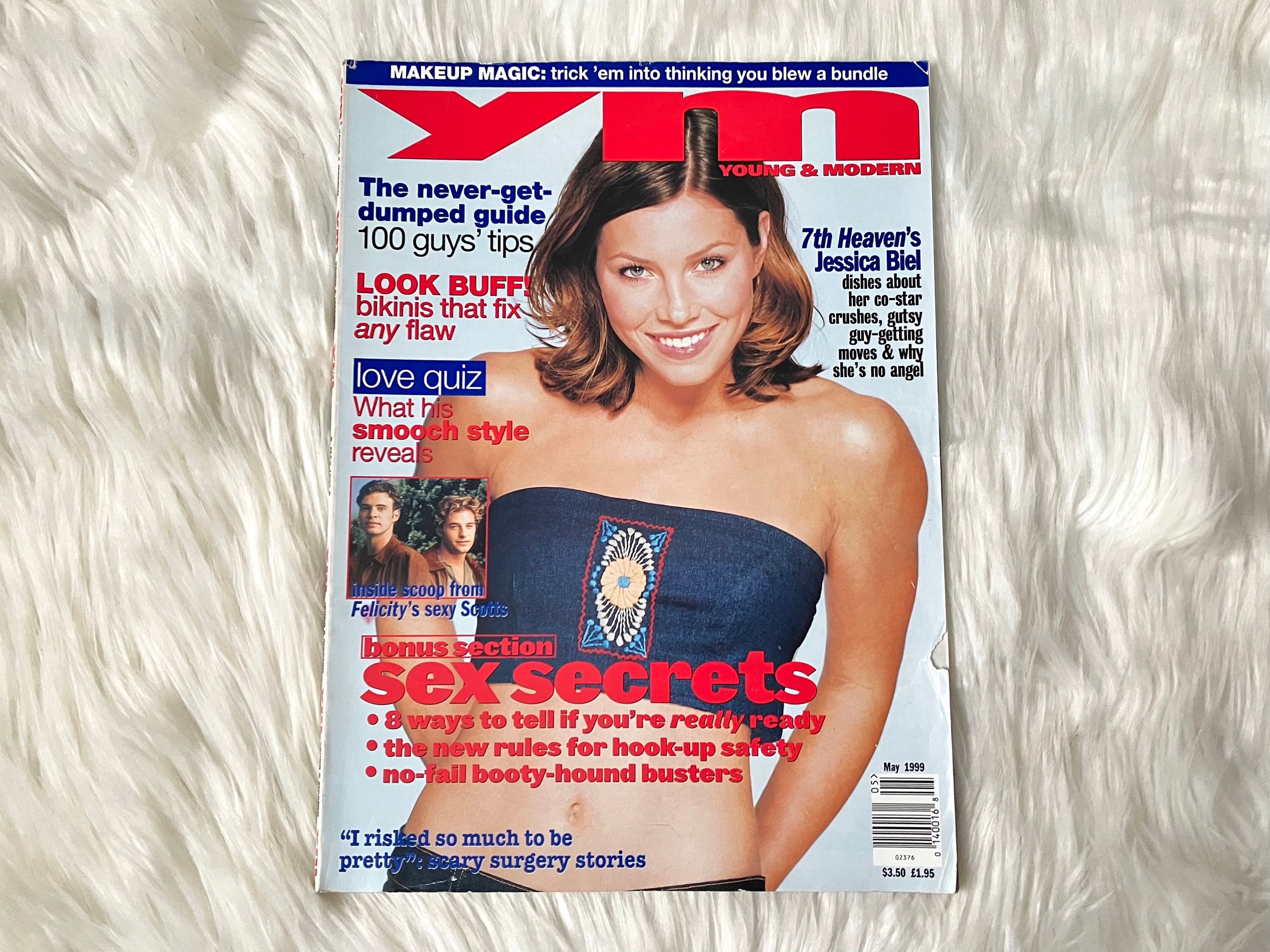The image displays an issue of the magazine YM (Young and Modern) from May 1999, laid out on a white and gray furry rug. The cover prominently features actress Jessica Biel with grayish-blue eyes and dark brown hair, wearing a distinctive blue denim bra adorned with a red-framed emblem in the center, and partially visible black belt. To her left, there's a smaller inset photo of Scott Foley and Scott Speedman, co-stars from the show "Felicity," with a green tree in the background.

The magazine's cover is packed with various headlines and article titles. At the top, there's a blue banner with white text reading, "Makeup Magic Trick: Trick ’em into Thinking You Blew a Bundle." Below, in red text, it states "YM Young and Modern." In blue text, it features "7th Heaven’s Jessica Biel," followed by black text detailing, "Dishes About Her Co-Star Crushes, Gutsy Guy-Getting Moves, and Why She’s No Angel." 

On the left side, in a blue box, it advertises a "Never Get Dumped Guide," complemented by "100 Guy Tips" in black. Nearby, in red text, it says "Look Buff: Bikinis That Fix Any Flaw," and in white text on a blue background, "Love Quiz," followed by "What His Smooch Style Reveals" in red.

Towards the bottom, against a light blue background, more announcements in red boxes include "Inside Scoop from Felicity's Sexy Scots," "Bonus Section," and "Sex Secrets" in bold letters. Bullet points under the latter promote articles like "Eight Ways to Tell If You’re Really Ready," "The New Rules for Hookup Safety," and "No-Fail Booty Hounds Buster." In the bottom left, it mentions, "I Risk So Much to Be Pretty: Scary Surgery Stories" in blue text.

The barcode is located in the lower right corner, with identifiers "350-195," "01400165" on the right, and "OS" with an arrow pointing up on the left, all set against a white background. The issue is priced at $3.50 in the United States and $1.95 in the UK.